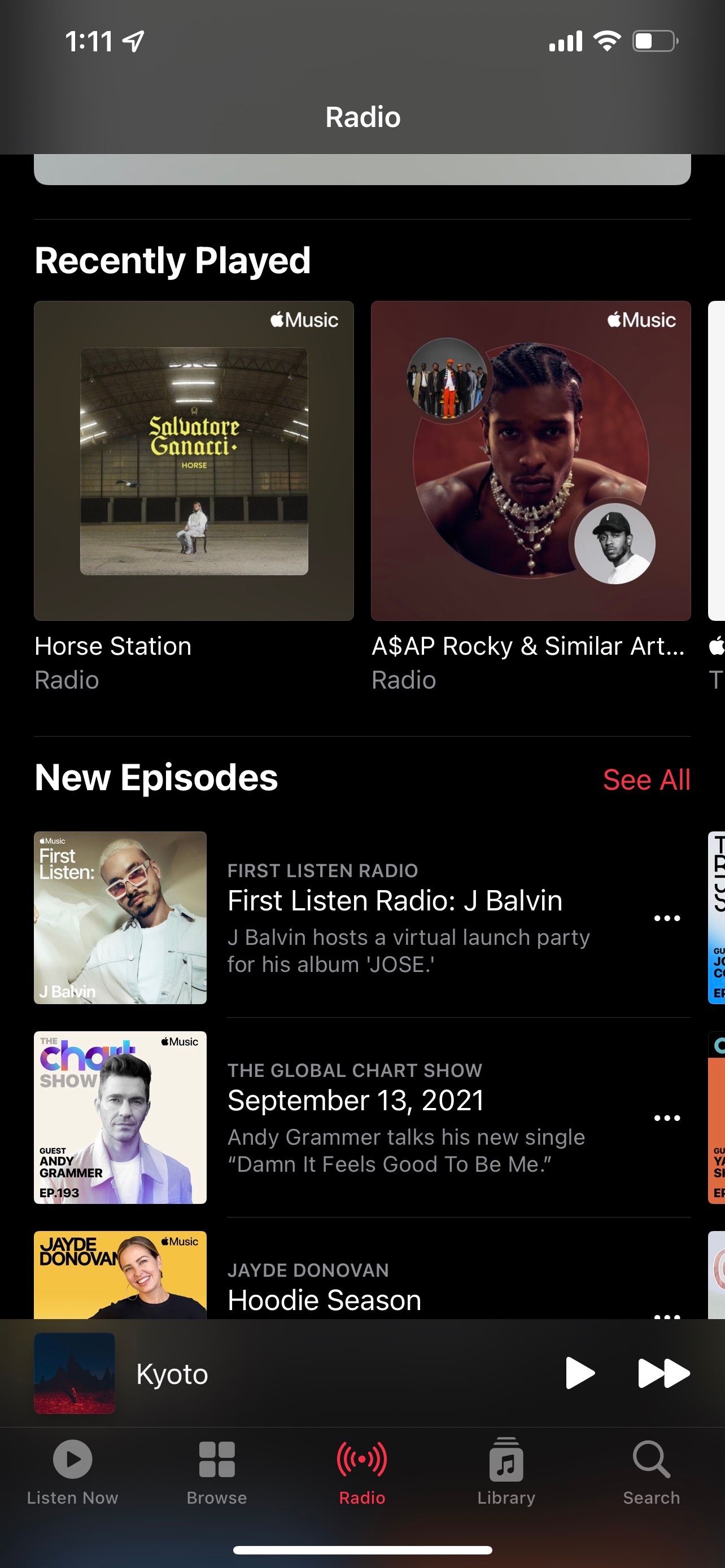Here is a cleaned-up and detailed caption for the provided image:

---

This image is a screenshot from the Apple Music app on a smartphone. The user is currently viewing the "Radio" section, as indicated by both the header text and the highlighted red icon at the bottom of the screen. The navigation bar at the bottom features five buttons: Listen Now, Browse, Radio (highlighted in red), Library, and Search – with the first two and the last two appearing in gray.

At the very top of the screen, the time is displayed as 1:11, and there are icons indicating the presence of another app, possibly a Maps or Navigation app, running in the background. The wireless connection, Wi-Fi, and cellular data icons all show full bars, while the battery icon is at half charge.

Just below the header, there is a "Recently Played" section displaying two albums: one with the cover art titled "Horse Station," and another by ASAP Rocky, partially obscured as "and similar art…". Below this section, there is a "Browse for New Episodes" section, with a prominent red button offering to "See All." Three episodes are visible: 

1. "First Listen: Radio with J Balvin."
2. "Global Chart Show," dated September 13, 2021.
3. "Andy Grammer talks about his new single, Damn It Feels Good to Be Me."

The third episode, "Jade Donovan - Hoodie Season," is also shown. At the very bottom of this section, the currently playing song is titled "Kyoto," with visible play and fast-forward buttons for media control.